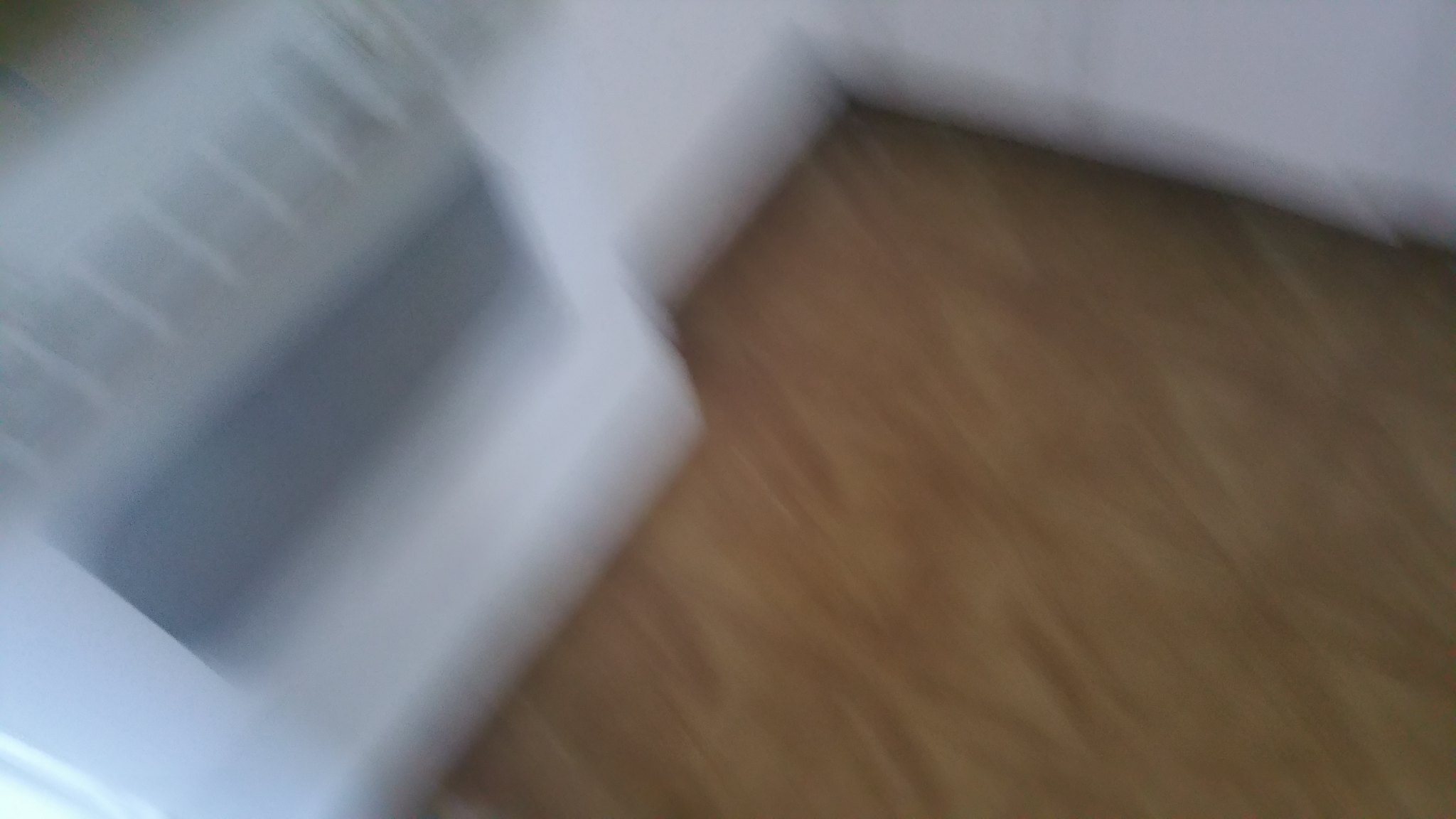The image is quite blurry and low in resolution, giving it a fuzzy appearance that suggests motion. The shape of the image is rectangular. On the right side, the dominant hue is brown, which appears to be a wooden floor. On the top right, there is a white platform that stretches to the left, resembling a kitchen counter. On the left side, within the white platform area, stands a white-gray item that appears to be a microwave, with what looks like an older style ice tray on top. The smooth, white kitchen counter contrasts sharply with the brown floor, and shadow details reveal a beveled edge and possible cabinetry doors beneath the counter. However, due to the blurriness, discerning additional objects or finer details is difficult.